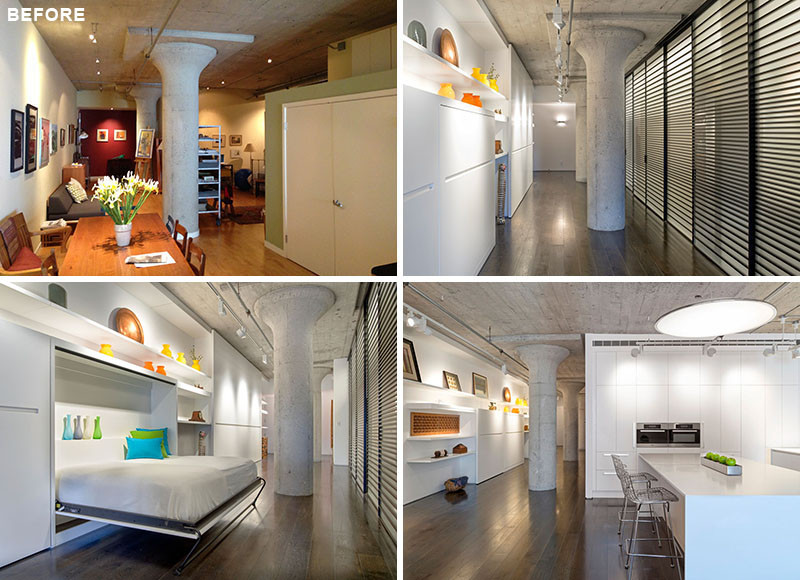This photo captures an impressive transformation of a small living space, depicted in a set of four images – two showcasing the 'before' state and two the 'after.' Originally, the room features a central white pillar, a wooden dining table, and wood flooring, along with a white double-doored cabinet positioned against a red back wall. The furniture occupies most of the space, accentuating the room's limited size. In the transformed 'after' images, the room has undergone significant changes. The flooring is updated to a dark gray, and the clutter is neatly stored away, with much of it hidden in innovative wall cabinets. One notable addition is a Murphy bed, adorned with red and green pillows, which seamlessly folds up to blend with the wall when not in use. Decorative elements like flower vases add a touch of style. On another angle, a white long table with two chairs sits adjacent to an oven embedded in the wall. Window blinds replace a previously visible cabinet, and the space now includes white shelves and a wall of pictures, giving it a modern and organized appearance. The remodel maximizes every inch, offering a functional, aesthetically pleasing living area despite the small size.